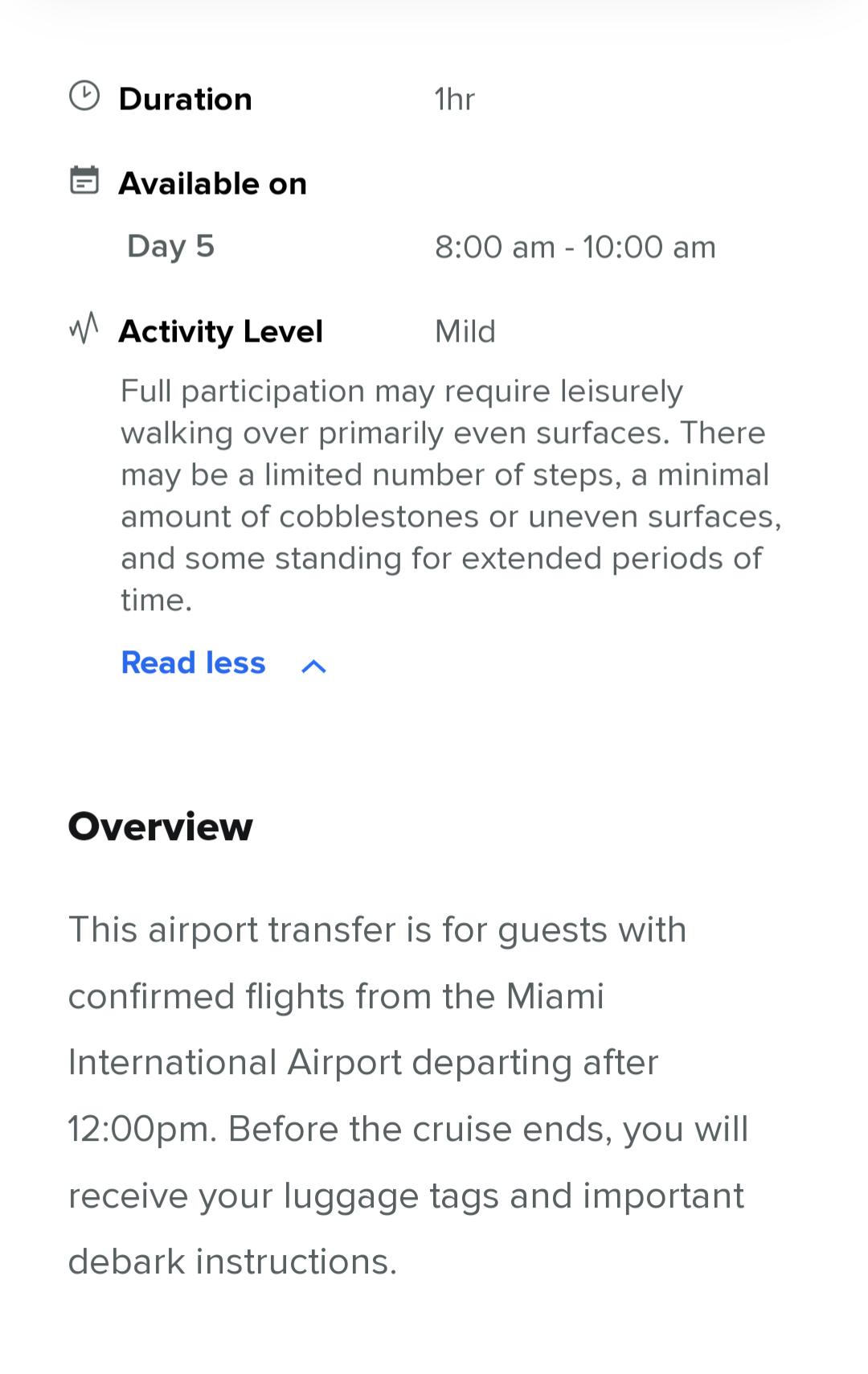This image is a mobile screenshot featuring a detailed itinerary. The image has a white background and consists of text framed without any visible borders. On the left-hand side of the image, there are categories labeled in bold, black font: "Duration," "Available On," and "Activity Level," each accompanied by a small icon. 

- **Duration:** Specifies "1 hour."
- **Available On:** Indicates "Day Five between 8 a.m. and 10 a.m."
- **Activity Level:** Classified as "Mild."

Underneath the "Activity Level" category, there is a detailed description that reads: 
"Full participation may require leisurely walking over primarily even surfaces. There may be a limited number of steps, a minimal amount of cobblestones or uneven surfaces, and some standing for extended periods of time."

Additionally, there is an option in blue font to "Read less," accompanied by an up arrow (⌃) symbol.

At the bottom of the image, under the "Overview" section, it states:
"This airport transfer is for guests with confirmed flights from the Miami International Airport departing after 12 p.m. Before the cruise ends, you will receive your luggage tags and important debark instructions."

The overall layout is text-centric with clear distinctions between categories, providing meticulously organized information for users.